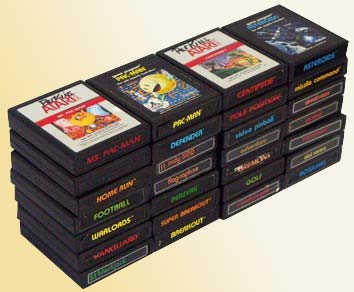The image features four stacks of vintage black Atari game cartridges, arranged in neat columns on a beige and light pink background. Each cartridge is adorned with colorful labels. Among them, one sports a white label with a red strip and a classic yellow smiley face, accompanied by the word "Atari" in red letters. Another cartridge highlights the iconic yellow Pac-Man character on a blue background with the title "Pac-Man" in prominent yellow letters. Additionally, there is a cartridge with a silver metallic hand and blue text. The vibrant labels showcase a mix of red, blue, orange, yellow, and green colors, providing a nostalgic glimpse into the array of classic games such as Pac-Man, Ms. Pac-Man, Centipede, Defender, Home Run, and Football. All the game cartridges are situated on a softly-colored, contrasting background that enhances their vintage charm.